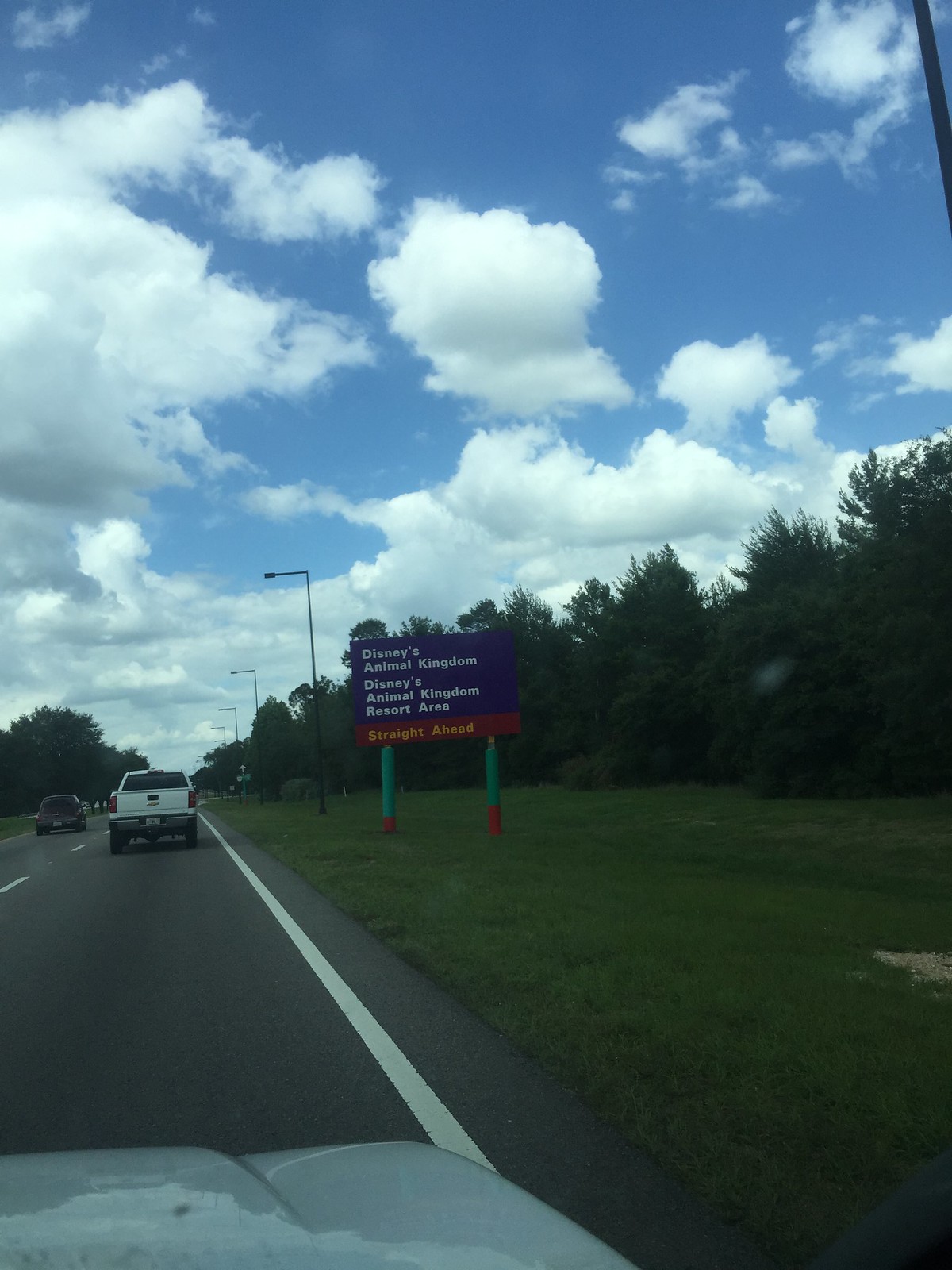This daytime photograph, taken from inside a vehicle, captures a scene with the light-colored hood of the car at the bottom. The well-maintained dark gray pavement of the road is clearly visible, punctuated by stark white lines. Directly ahead, a white pickup truck travels along the road. Off to the side, there's a stretch of short, green grass leading up to a sign. The sign is supported by green and red poles, with a red base displaying the word "Straight Ahead" in white text. Above that, on a royal purple background, white font announces "Disney's Animal Kingdom" and "Disney's Animal Kingdom Resort Area." Behind the sign, lush green trees stand tall, contrasting with several black light poles. The sky above is a brilliant blue, dotted with fluffy white clouds. In the distance, other vehicles can be seen making their way along the road.